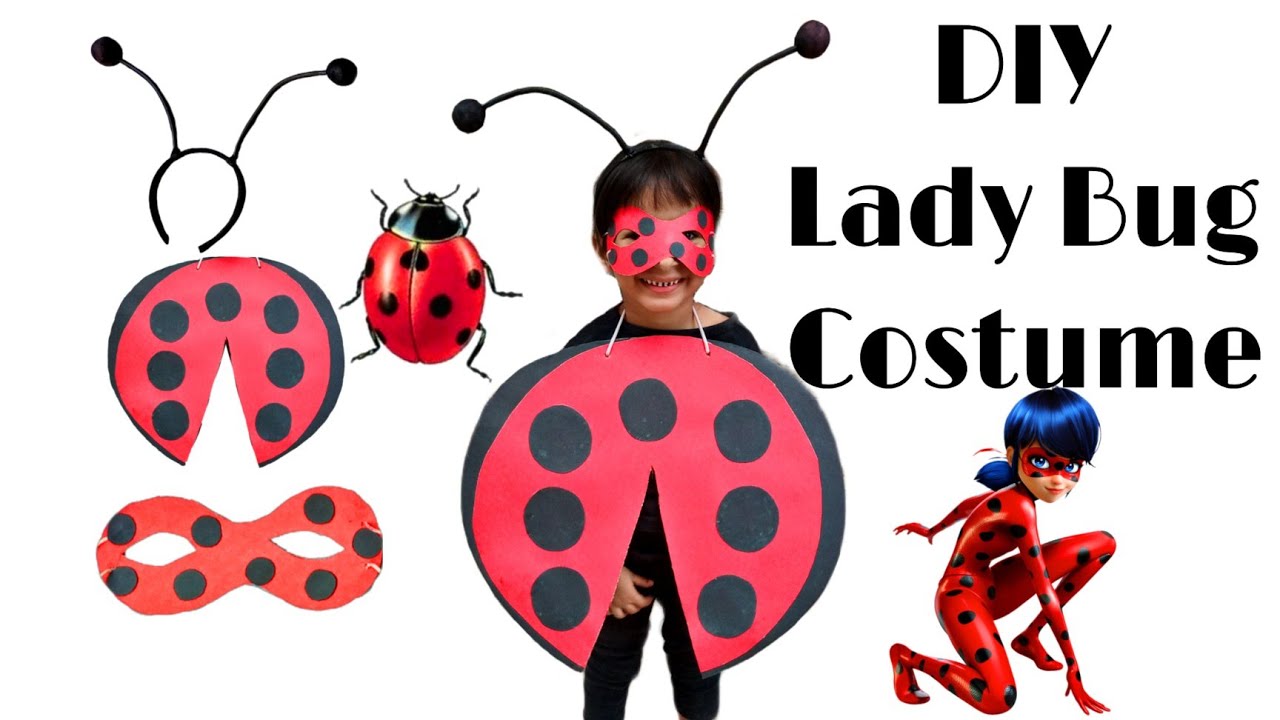The image displays a young child, excitedly smiling while showcasing a DIY ladybug costume. The costume, crafted from cardboard, features a red body with black spots that hangs from the child's neck. Complementing the outfit is an eye mask adorned with black dots and a headband decorated with ladybug antennae. The child is dressed in black pants and a black shirt, emphasizing the vibrant costume. To the right of the child is the text "DIY Ladybug Costume," indicating the image's theme. Surrounding the child are detailed instructions and parts needed to create the costume. Additionally, there is a depiction of a ladybug and an animated character dressed in a sleek, red jumpsuit with black polka dots, blue wig, and red mask. This intricate layout serves as both an advertisement and a guide for creating a charming ladybug ensemble at home.